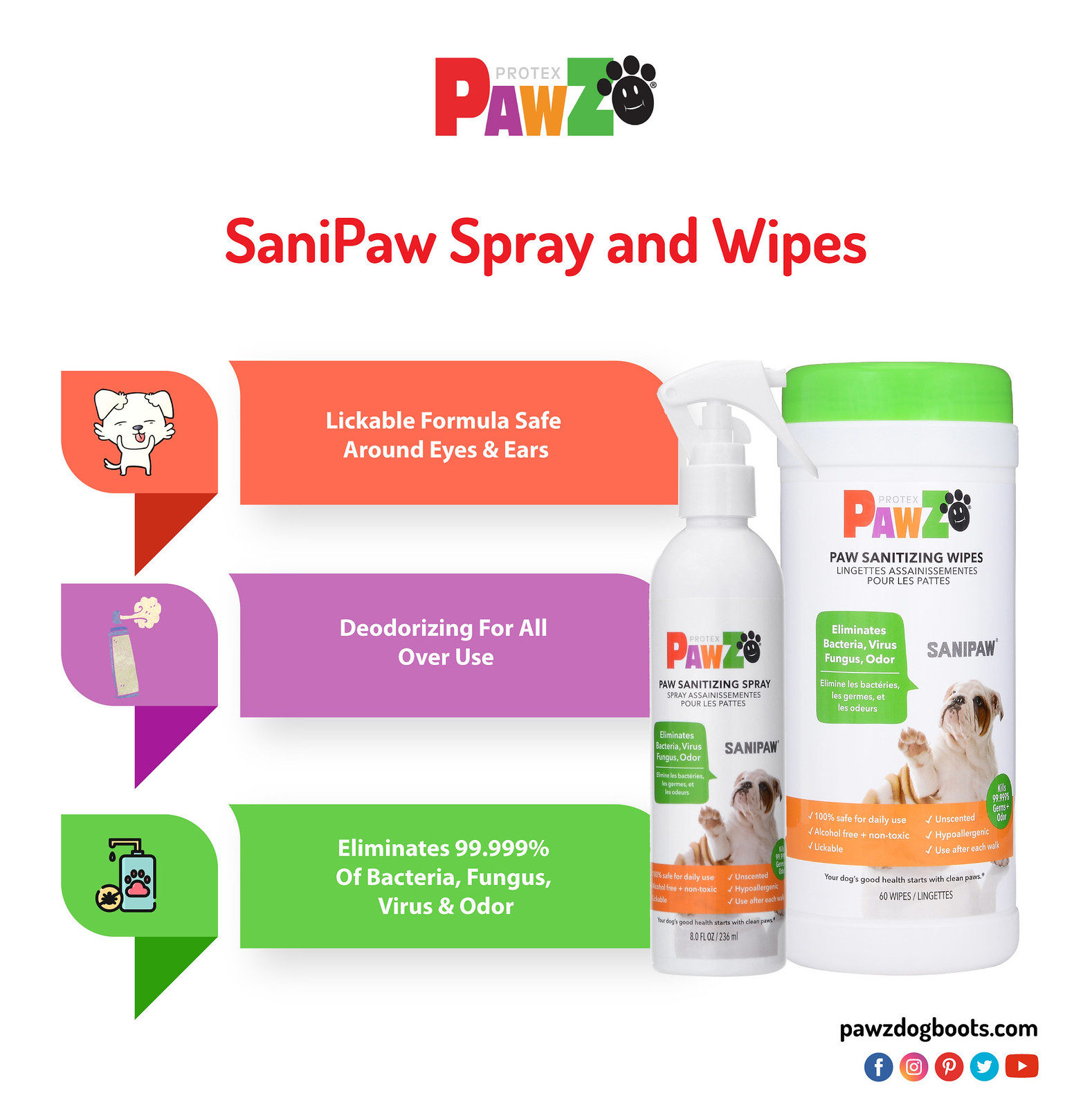This image is an advertisement for Pro-Tex Paws' sanitizing pet product, Sani Paw Spray and Wipes. At the top of the advertisement, the logo reads "PAWZ" with a stylized paw print featuring a smiley face. The "P" is red, the "A" is purple, the "W" is orange, and the "Z" is green and larger than the "A" and "W," matching the size of the "P." Below the logo, in large red letters, it says "Sani Paw Spray and Wipes."

Down the left side, three colorful banners provide key information: 

1. A red banner that reads "Lickable Formula Safe Around Eyes and Ears," accompanied by an image of a happy cat.
2. A purple banner that reads "Deodorizing for All Over Use," with an icon of a spray can.
3. A green banner stating "Eliminates 99.999% of Bacteria, Fungus, Virus, and Odor," next to a dripping sanitizer icon.

To the right of these banners, the actual products are displayed: 

- A spray bottle labeled "Paw Sanitizing Spray," featuring a cute white and brown bulldog with its right paw raised. There is also a green speech bubble above the bulldog.
- A cylindrical container of wipes labeled "Paw Sanitizing Wipes," capped with a bright green lid. This also features the same bulldog and speech bubble.

At the bottom left, the website "PawsDogBoots.com" is listed, followed by icons for social media platforms including Facebook, Twitter, Instagram, Pinterest, and YouTube.